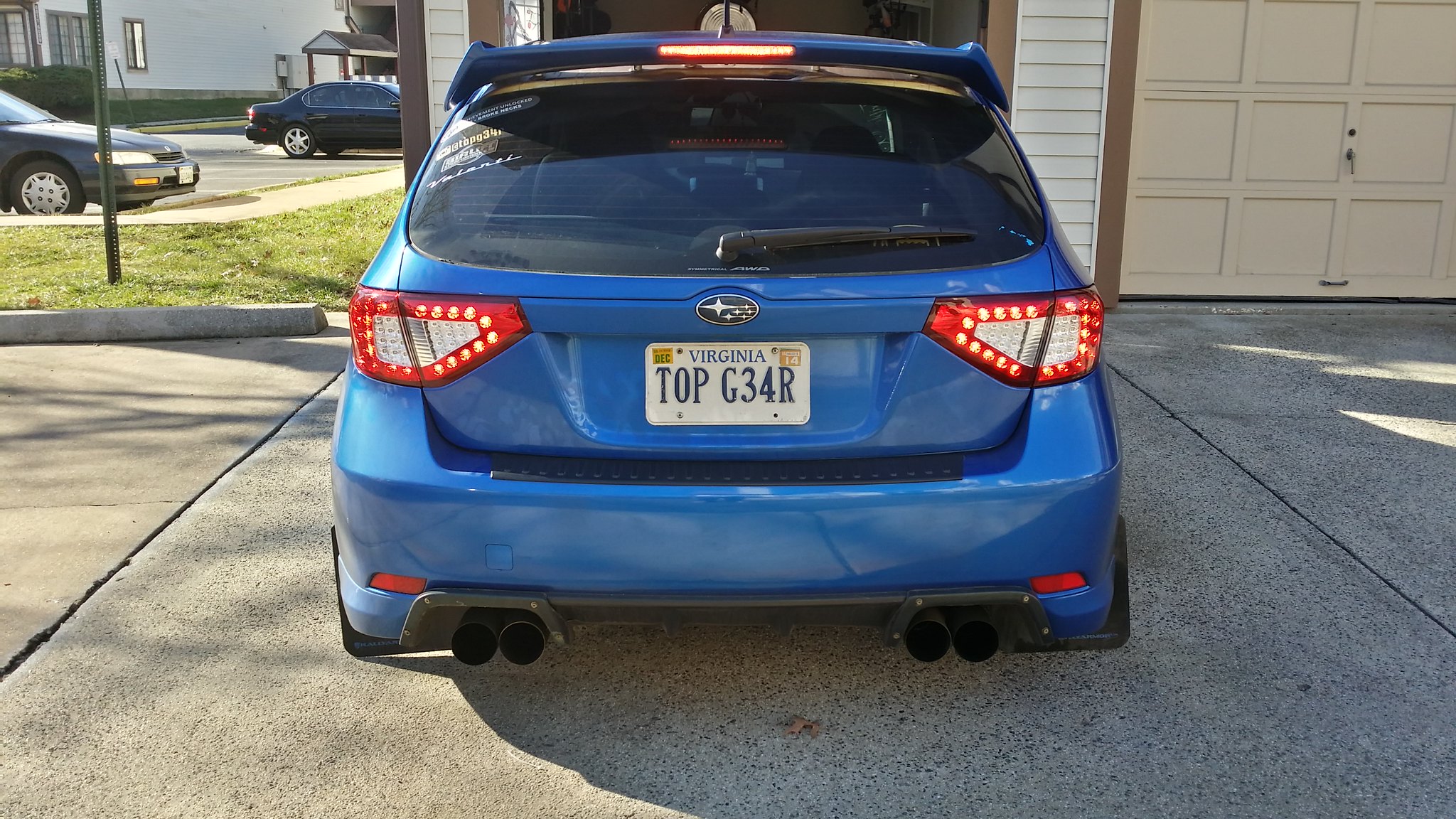This photograph captures a bright royal blue Subaru parked in a gray paved driveway in front of a partially open garage door, with white siding and dark brown trim. The other garage door next to it is tan-colored. The vehicle, a newer model indicated by its dual exhaust pipes and advanced taillights featuring red accents and dotted illumination, sports a Virginia novelty license plate reading "T0P G34R," mimicking "Top Gear." Interestingly, the car's brake lights are on, suggesting someone might be inside. In the background, there are visible features such as additional cars parked in designated spots, an entranceway, and another nearby building with what appears to be mailboxes, hinting at a townhouse or apartment complex setting.